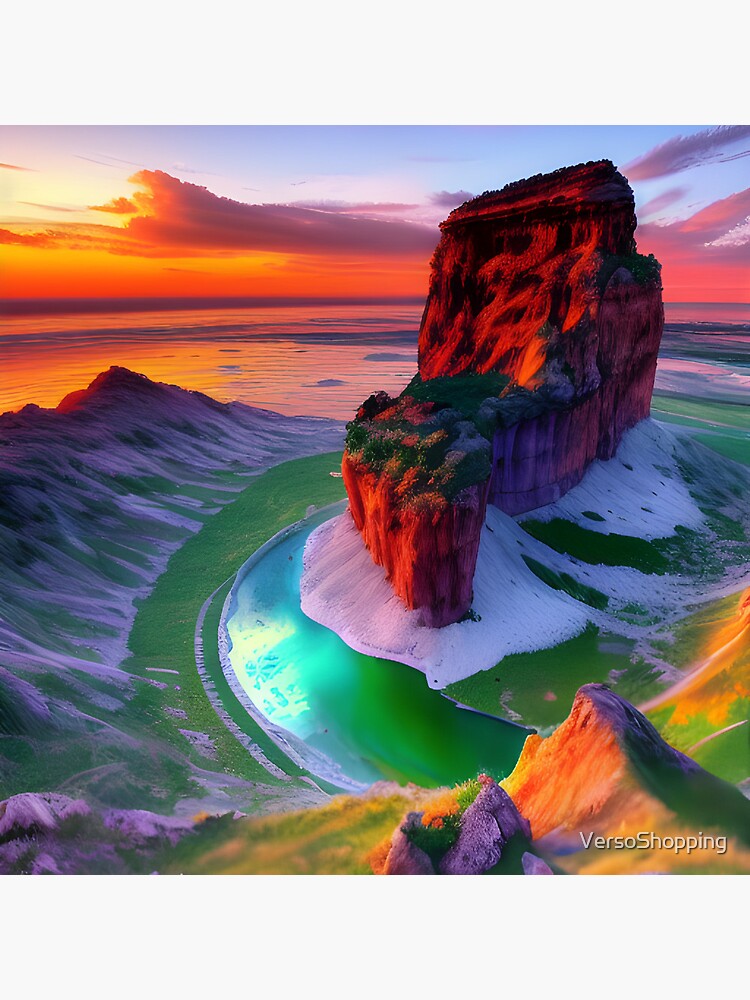The image portrays a surreal, likely computer-generated scene of a mountainous structure situated on an island-like formation in the middle of an ocean. The focal point is a striking mountain face, predominantly red with touches of brown, orange, and green foliage clinging to its surface. This mountain is set against a sweeping, vibrant sunset marked by purplish clouds blending into hues of pink, yellow, and a brilliant orange. The sky casts a warm glow, enhancing the surreal nature of the setting. 

The water surrounding the structure transitions from a deep green to a mixture of whites and blues, with small ripple waves evolving into larger waves that appear to crash around the island. At the base of the mountain, snow can be seen, contrasting with the green foliage and the colorful hues of the structure itself.

In addition to the main mountain and its surrounding seascape, the foreground features additional rocky landscapes in shades of red, green, gray, and white. Further details, such as the green grass in the background and additional mountain pieces to the right, add depth and complexity to the scene. The bottom right corner of the image contains the text "Verso shopping" in white, suggesting perhaps a subtle or intentional branding within this intricate, abstract depiction of a natural yet fantastical environment.